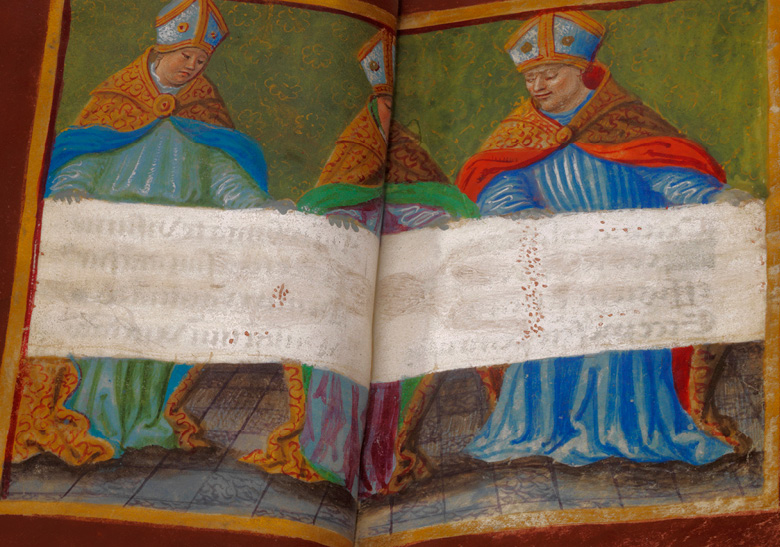The image showcases an aged, historical text, likely an illuminated manuscript or tapestry, featuring three ornately dressed religious figures, possibly cardinals or saints. The characters are positioned across an open book, with vibrant maroon-red and yellow-orange borders framing the scene. The background is a dark, sketchy green with hints of yellow light filtering through. The central figure, partially obscured due to the book's spine, dons a green robe beneath a gold-orange vestment and a blue-orange hat. To the left, another figure in a blue robe and gold vestment wears a cardinal's hat, his gaze directed downward. The right figure is similarly attired in a red cloak, blue gown, and ornate hat, also looking towards the center. All three figures are focused on a large, rectangular white scroll or paper that spans both pages, featuring faded, nearly unreadable text. The rich, detailed vestments and the positioning of the figures suggest a significant religious or ceremonial depiction, framed by a detailed maroon and yellow-orange border indicative of the period's artistic style.